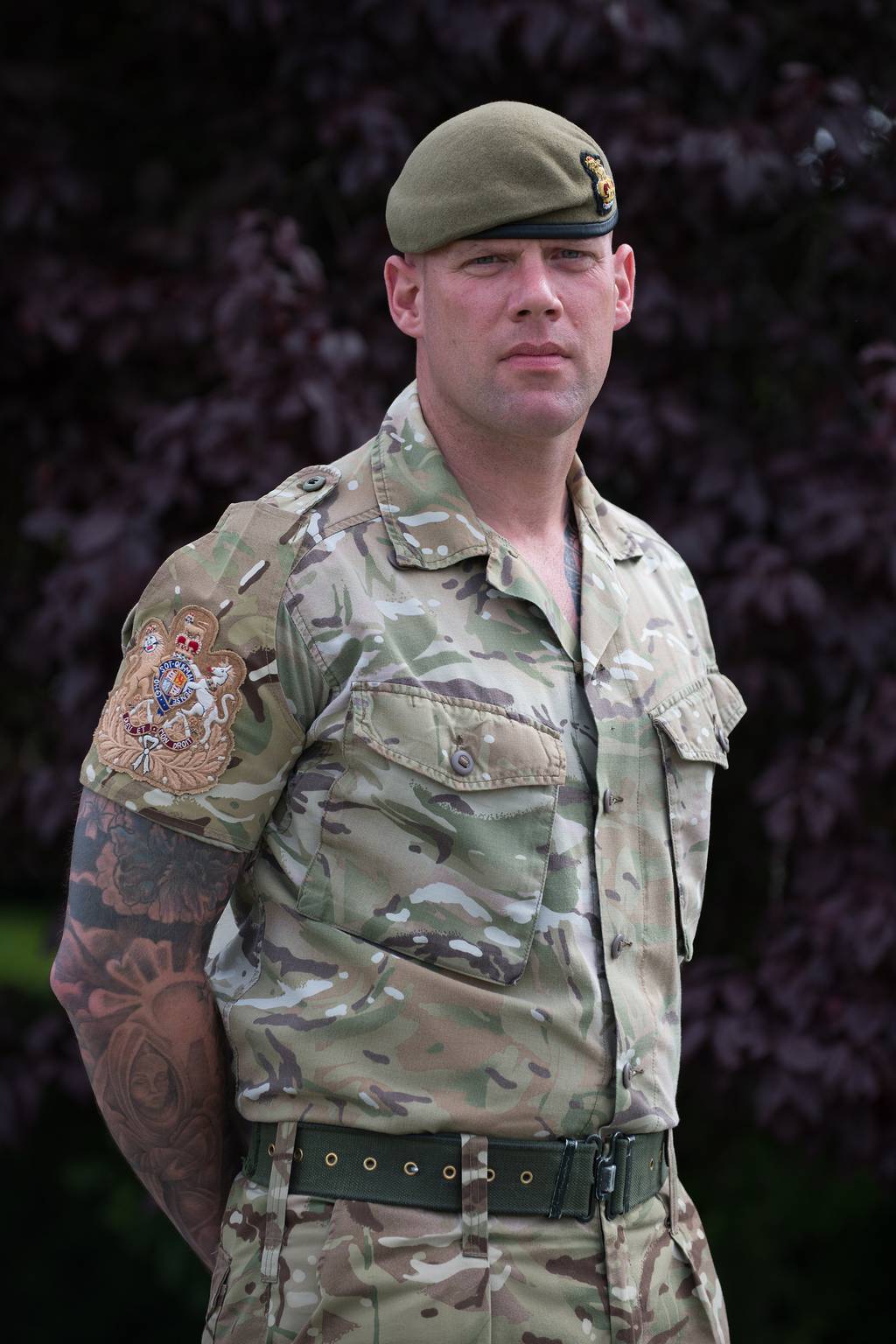This image features a tall, clean-shaven Caucasian military man dressed in classic camouflage army fatigues. His outfit includes a short-sleeved top and matching camouflage pants, secured with an olive-green belt. On his head, he wears an olive-green beret with a black band at the bottom, adorned with a golden crest emblem on the side. His right shoulder bears a detailed patch depicting a white horse, a golden lion, a crown, and a shield with some leaves at the bottom, likely indicating his regiment or division. His left arm displays a full sleeve of intricate black tattoos, featuring what appears to be a religious figure with a cloak and a sun motif. The background is filled with purple foliage and flowers, enhancing the overall impression of a clear, bright day. His head appears to be shaved under the beret, as no hair is visible beyond its edge.